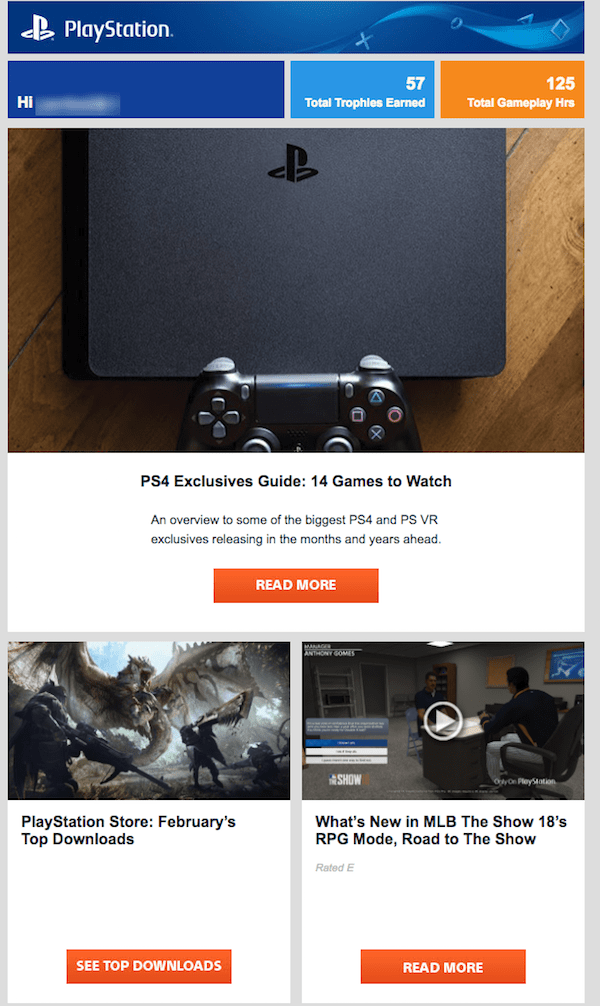The image appears to be a screenshot taken from a phone, indicated by its vertical, rectangular shape. The screenshot is bordered by slim gray edges on the sides, with a deep dark blue border adorning the top. This upper border has a wavy design on the right side, featuring PlayStation symbols in its center - an X, an O, a triangle, and a square. 

In the upper left corner, the white PlayStation icon and the word "PlayStation" are prominently displayed next to another thin light blue line. Below this line, extending halfway across the screen in the bottom left corner, sits a long dark blue rectangular tab with the greeting "Hi," followed by a blurred word.

At the bottom of the screenshot, a light blue tab displays in white text "Total Trophies earned: 57." Directly below it, an orange tab reads "Total game hours: 125."

Central to the image is an overhead picture of a black PlayStation console with a controller, situated on a wooden table. The background beneath it is completely white, featuring bold black text that proclaiming "PS4 Exclusive Guide: 14 games to watch." This is followed by two lines of text providing additional information about upcoming games, and an orange tab highlighting "Read More" in white lettering.

A thin gray border runs through the center of the screenshot, dividing it into two sections. On the left side, there's an image of a person fighting a dragon, situated above the text "PlayStation Store February's top downloads," followed by a gap and an orange tab stating, "See top downloads."

On the right side, a person is seen sitting at an office desk with a play button in the center of the image. Text below says, "What's New in MLB The Show 18," followed by "RPG mode, Road to Show." At the very bottom, another orange tab reads "Read more" in white text.

The extensive use of PlayStation branding and the detailed information suggests that this is a promotional screenshot, possibly from an official PlayStation app or service.